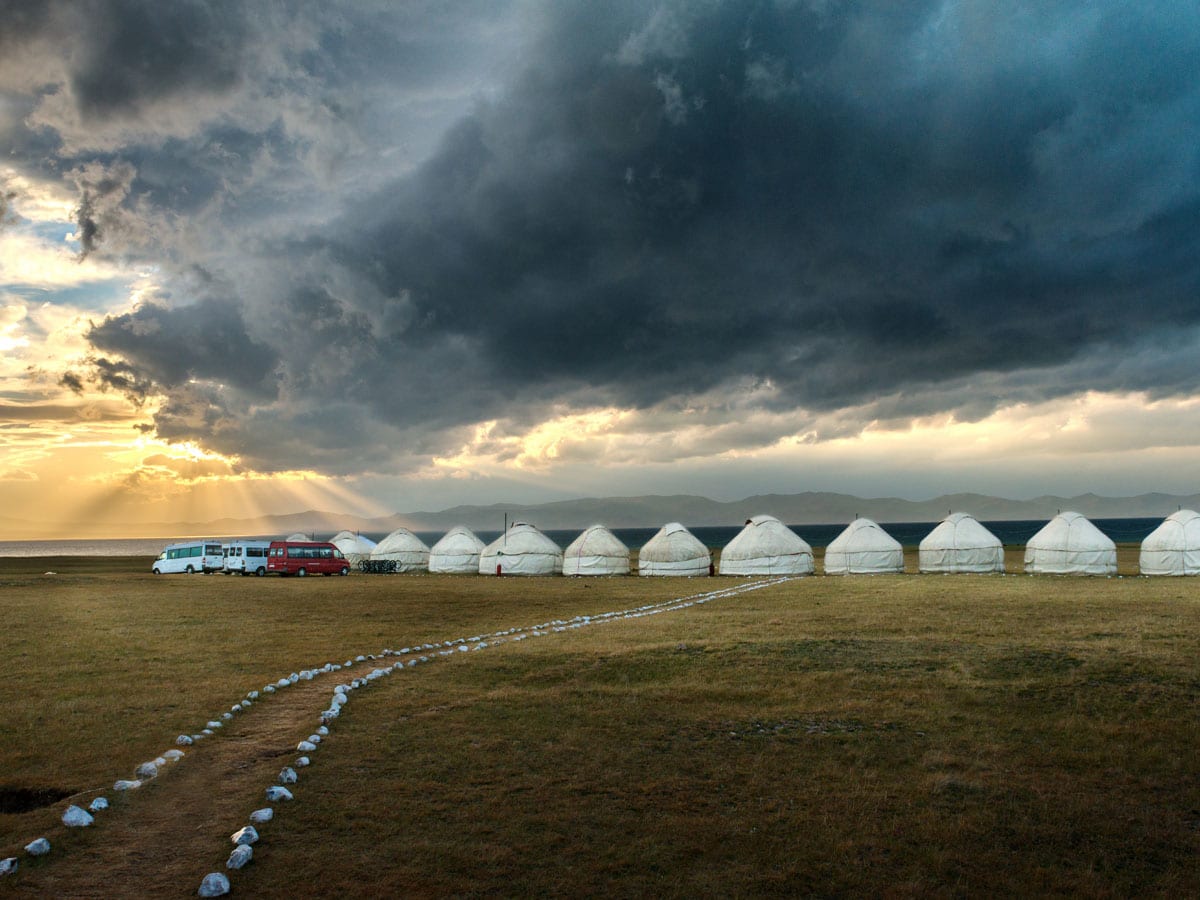The square picture depicts an outdoor scene on a prairie-like landscape under a dramatic sky. The upper two-thirds of the image showcase a very cloudy sky with layers of dark gray clouds mingling with lighter ones, creating an ominous atmosphere suggestive of an impending storm. However, towards the left side of the image, rays of sunshine break through, revealing patches of blue sky and illuminating the scene below. In the background, an outline of distant mountains or hills is faintly visible.

Dominating the mid-ground of the image are 10 to 15 round, conical white tents arranged in rows from the right side to about three-fourths of the width of the photo. These tents contrast starkly with the short grassy field that covers the rest of the land. To the far left, in front of the tents, are three passenger vans—two white and one red—parked in a loose cluster. A narrow, rocky walkway starts at the lower left corner, cuts across the grass, and weaves between the two central tents, guiding the viewer’s eye into the scene. The overall composition creates a balanced yet dynamic depiction of a campsite set against a strikingly moody sky.